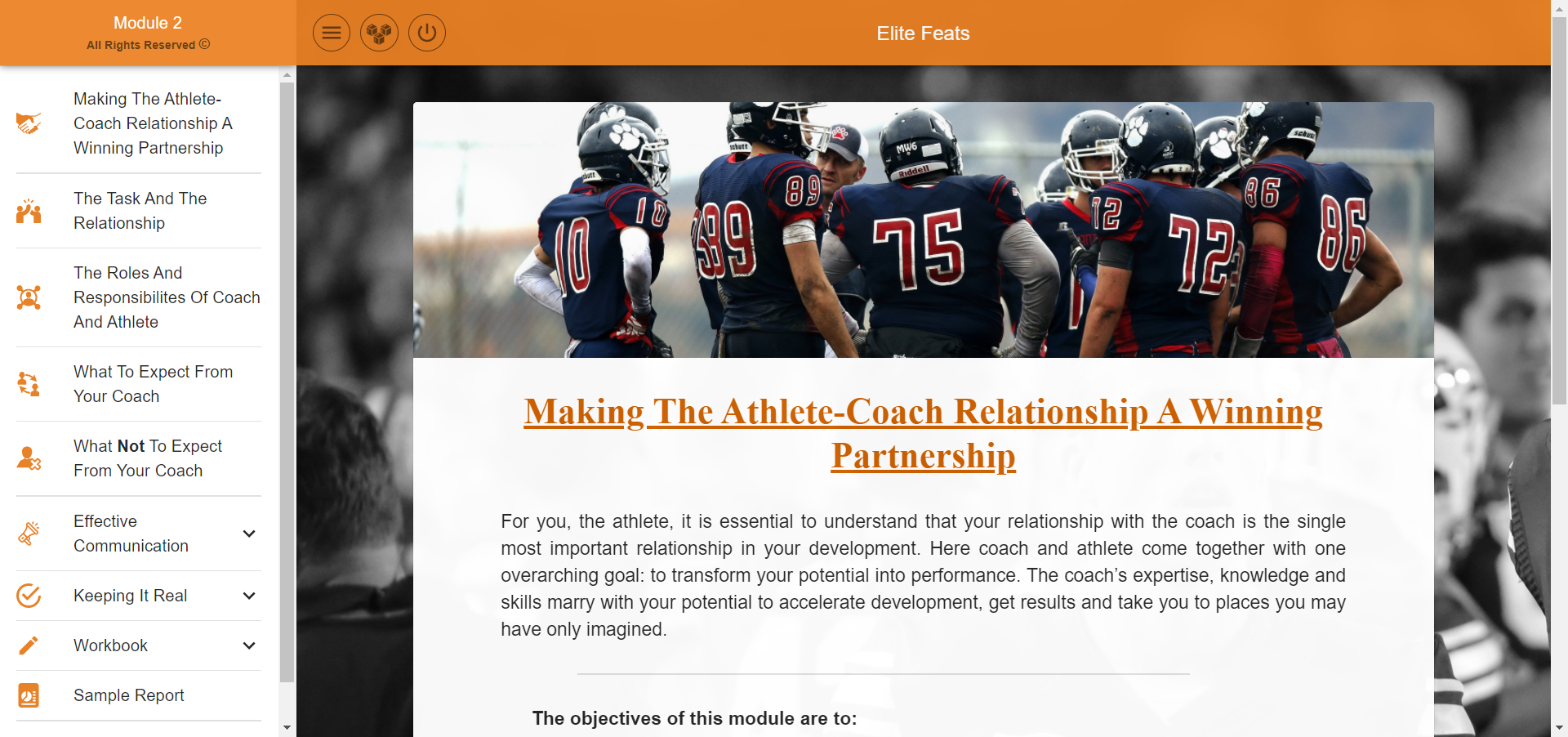The image is a screenshot from a webpage dedicated to an online course. The top border of the page is a muted burnt orange, within which the title "Elite Feeds" is prominently displayed in white text. The central section, occupying around three-quarters of the screen, features a banner at the top showcasing the backs of football players. They are donning blue uniforms, with their jersey numbers highlighted in brick red and outlined in white. 

Directly beneath this banner is a white rectangle containing the course title, "Making the Athlete-Coach Relationship a Winning Partnership," written in burnt orange font and underlined in the same color. Following the title, there is a course description in light gray text, emphasizing the vital nature of the athlete-coach relationship, stating, "For you, the athlete, it is essential to understand your relationship with the coach is the single most important relationship in your development." The description continues further, but is truncated in the image. 

At the bottom of this section, introductory text reads, "The objectives of this module are: and then the text is cut off. On the left side of the page, a sidebar presents a structured outline of the course's highlights and modules. Listed topics include "Making the Athlete-Coach Relationship a Winning Partnership," "The Task and the Relationship," "The Roles and Responsibilities of Coaches and Athletes," among other segments, suggesting a comprehensive approach to understanding and fostering the athlete-coach dynamic.